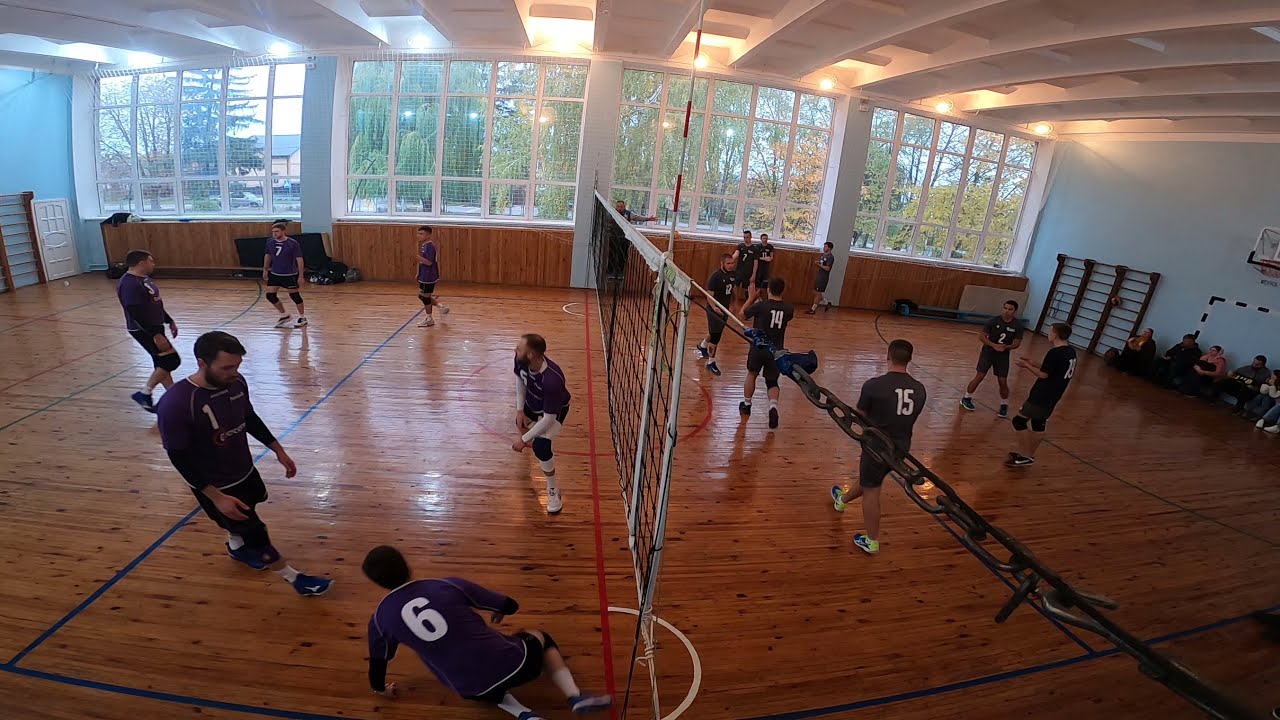The image captures a lively volleyball match taking place in an indoor gymnasium. The court's floor is a reddish-brown hardwood with blue, red, and white striping. At the center of the court is a volleyball net with white borders, held up by red and white poles attached by a chain. Six players on each team are positioned on either side of the net, dressed in long sleeve navy shirts, black shorts, and white shoes, with some players standing and others interacting or diving for the ball. Their jerseys feature white numbers. Spectators are seated along the perimeter of the court, watching the game unfold. The gym's ceiling is white, featuring a beam design with recessed lighting of various temperatures. Large windows framed in white line the far wall, partially covered by protective screens, and daylight streams in, offering a view of trees outside. The walls surrounding the gym are painted a very light blue.